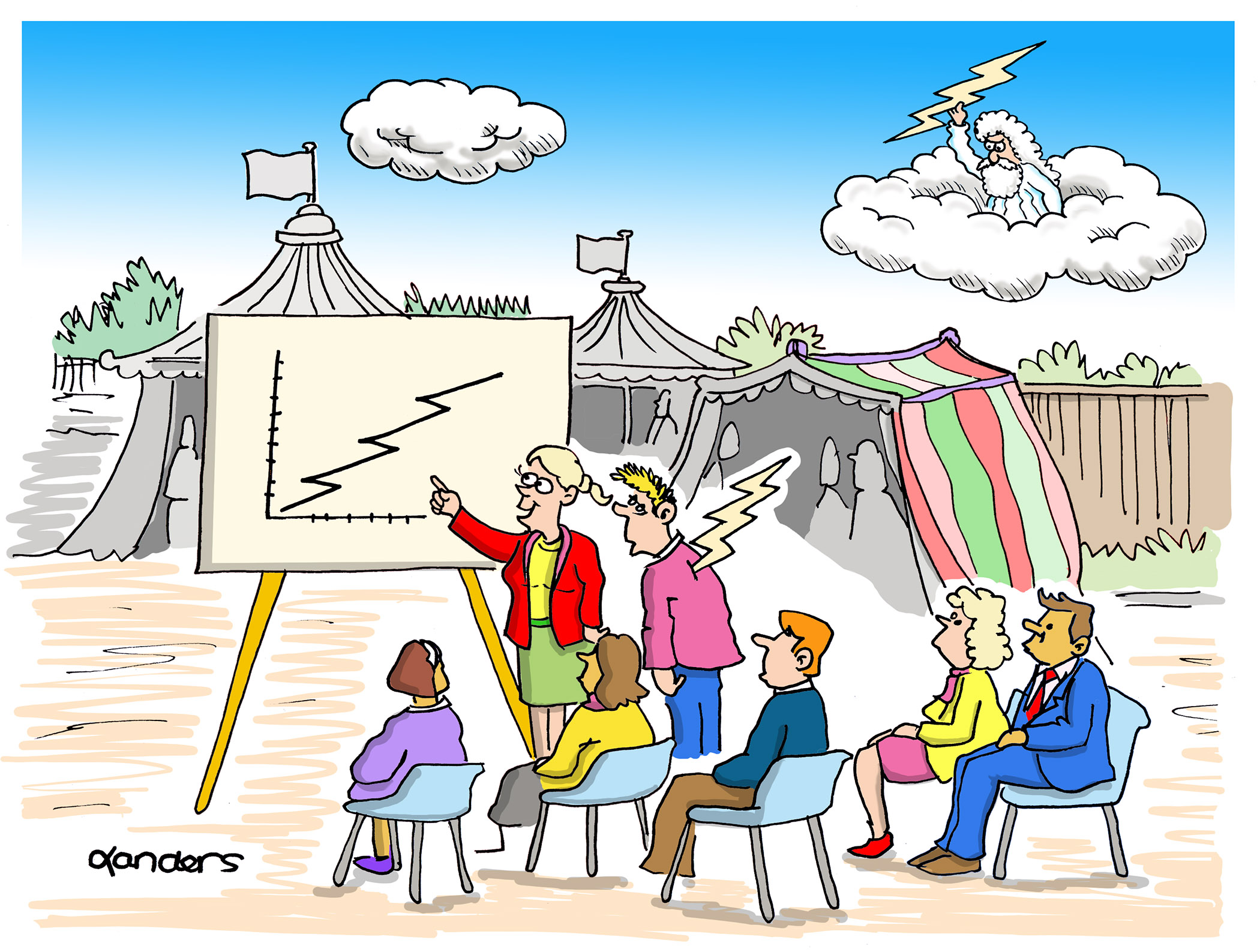This comic-style illustration depicts a group of individuals seated in plastic chairs, engaged in a meeting and all gazing intently at a large chart. The chart, which shows a lightning bolt-shaped line graph trending upwards, is being pointed at by a smiling woman. She stands beside a male colleague who has a lightning bolt striking from his back. The scene is set against a backdrop of circus tents, with trees visible in the distance. Hovering above them in a cloud, a robed figure with long white hair ominously wields a lightning bolt, poised to hurl it downwards. The atmosphere blends the mundane with the surreal, creating a strikingly bizarre yet detailed visual narrative.